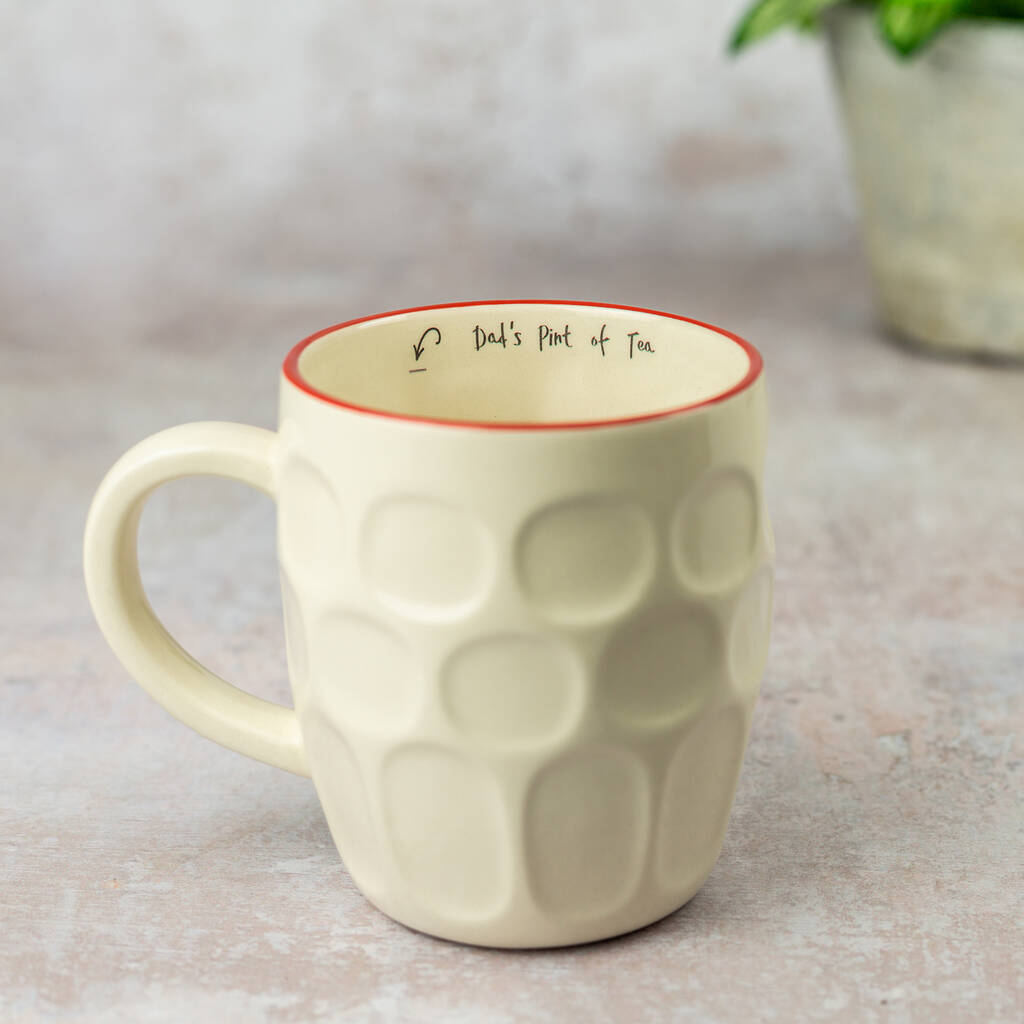This image showcases a detailed, textured white teacup with a pinkish-red brim, prominently centered on what appears to be a stone table or countertop. The teacup, adorned with an indented pattern resembling circles and ovals, features black lettering on the inside near the lip that reads "Dad's pint of tea," accompanied by a playful, curving arrow pointing towards the text. To the upper right of the composition, there is a potted plant with green leaves in a white vase, adding a touch of natural greenery to the scene. The background includes shades of green, white, gray, red, and black, contributing depth and context to the overall setting. The teacup's handle is positioned to the left, indicating it is ready to be picked up with the left hand. This real photo captures a moment of homely charm and personal touch.